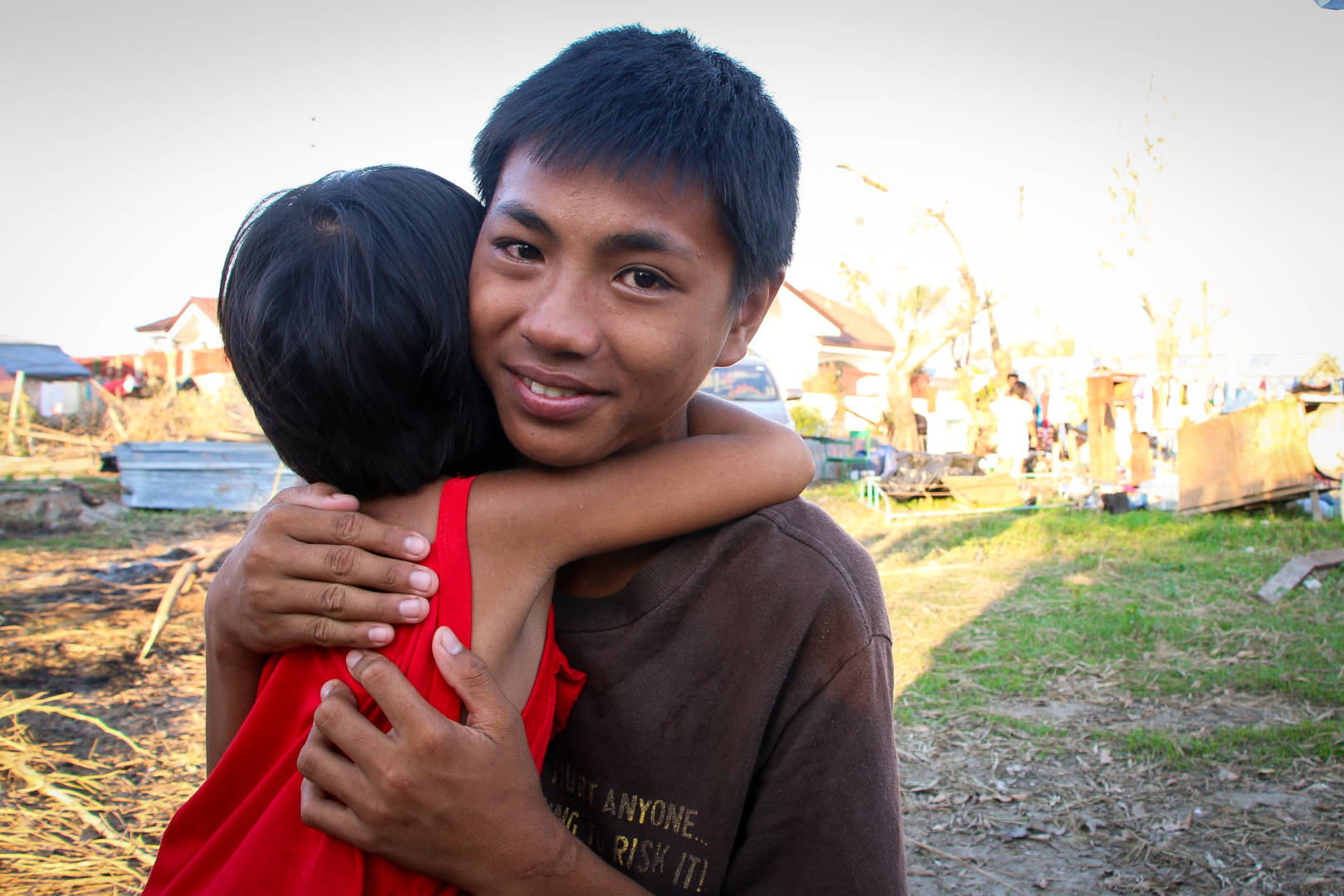This vibrant outdoor color photograph features two children of Southeast Asian descent sharing a heartwarming embrace. The older boy, positioned centrally and facing the camera with a wide, joyful smile, has short black hair styled in a bowl cut and tan skin. He is dressed in a brown t-shirt and radiates warmth as he hugs a smaller child. The younger child, who also has short black hair and tan skin, is wearing a red sleeveless tank top and has his arms wrapped lovingly around the older boy's neck. The setting appears to be an outdoor residential area with grassy patches, scattered stones, branches, and signs of a possibly cluttered neighborhood environment, including visible houses and buildings that are partially illuminated. Shadows suggest it is late afternoon, contributing to the warm, serene atmosphere of the scene.